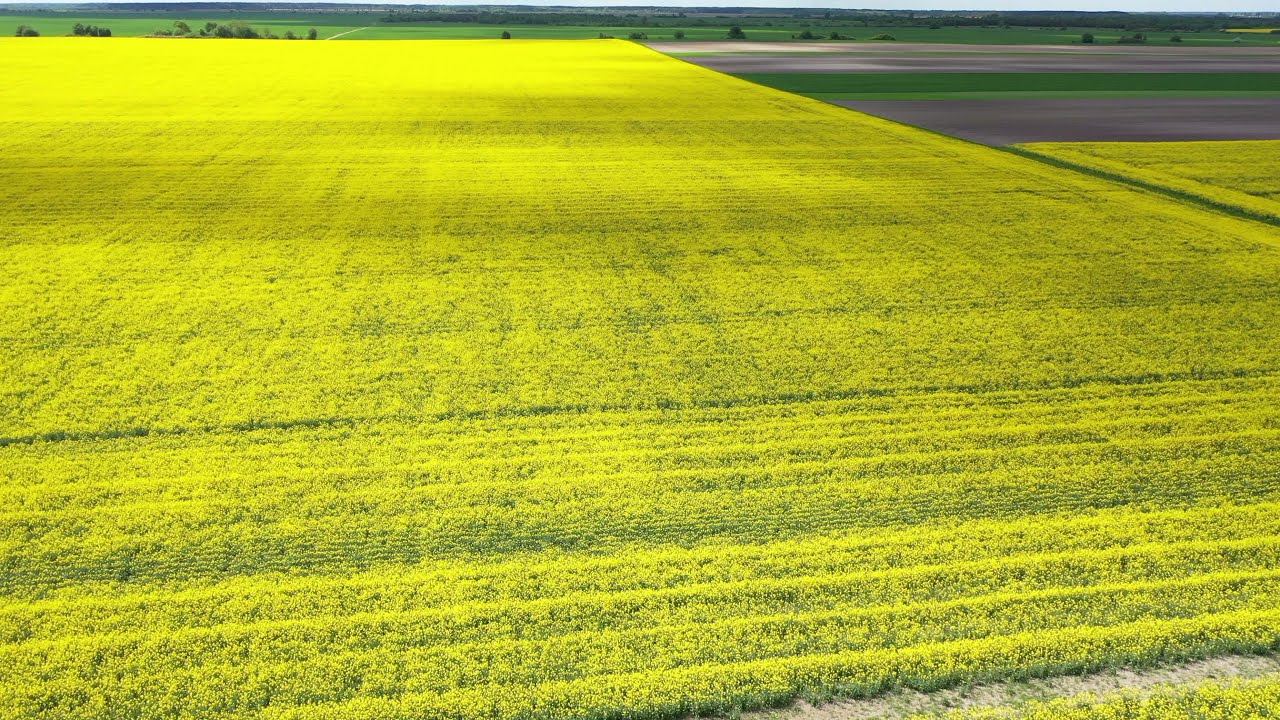The image captures a vast, rectangular field blanketed with small yellow flowers, likely crops such as sunflowers or rapeseed. These uniform flowers create a stunning, consistent pattern, almost as if the field were rolled out like a vibrant carpet. The flowers transition from dark green at the roots to bright yellow at the tips. Overall, they occupy about 85% of the image, with subtle shading from clouds casting light shadows across parts of the field. In the background, various patches of land create a mosaic of colors; there's a small sliver of green grass and grayish dirt on the upper right-hand side, indicating possibly harvested areas. As the field extends towards the horizon, it meets a thin line of bushes and trees, with more fields visible beyond. The land is generally flat, adding to the serene and expansive feel of the scene.